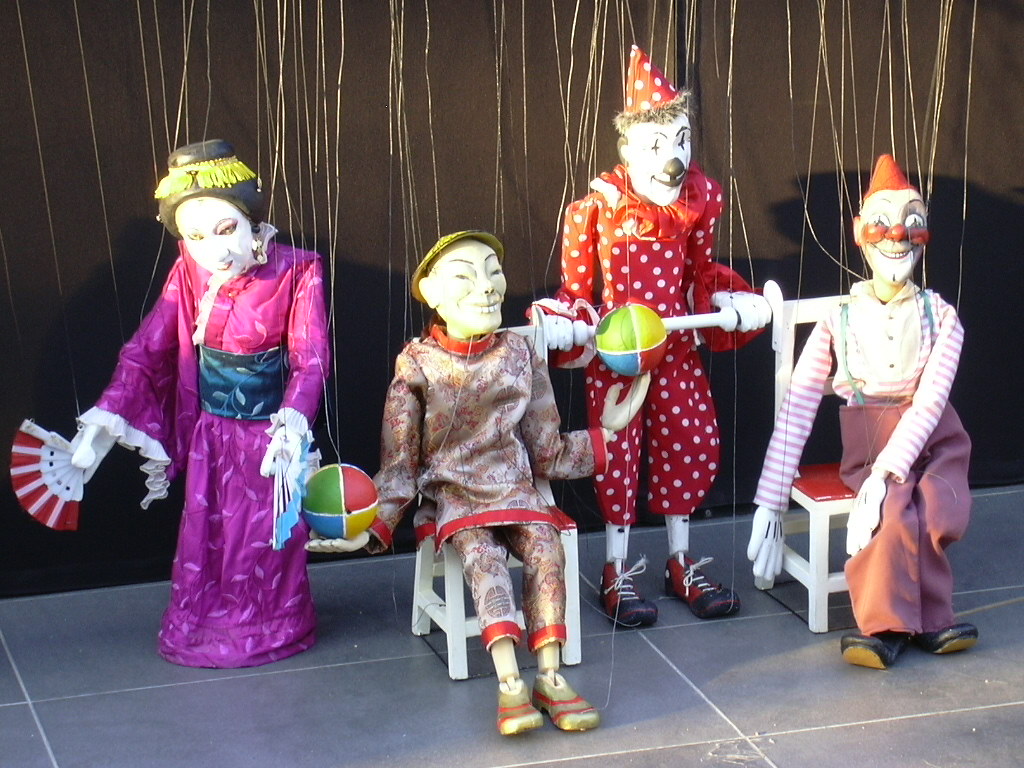The image depicts a detailed and ornate miniature stage with a gray tiled floor and a black fabric backdrop representing a curtain. On this custom stage, there are four meticulously crafted marionette dolls, each adorned with traditional Japanese-style clothing and vivid clown makeup, bringing an eclectic cultural fusion to life.

The marionette on the far left resembles a geisha, dressed in a purple or violet kimono, with a large blue band and white ruffles around the hands. She holds a fan and has black hair highlighted with yellow, adorned with very white makeup. Next to her stands a juggler marionette, attired in matching silk-like prints that mimic pajamas, complete with a yellow hat and shoes that match his outfit. He holds two brightly colored balls with red, green, blue, and yellow segments divided by white lines.

The third marionette, positioned to the right of the juggler, is a classic clown. This figure is outfitted in bright red clothing with white polka dots and wears a corresponding party hat. His face is painted with white makeup, featuring a black nose and crosses on the eyes, likely meant to give an expressive, exaggerated look.

Finally, the marionette on the far right sits on a stool with a round seat. He is dressed in baggy, purplish pants, black clown shoes, a black and white striped shirt, and white gloves. His face sports a big red nose, red cheeks, and white face paint complemented by a small red party hat. This detailed marionette stage setup, complete with intricate strings attached to the dolls, captures a whimsical and slightly eerie scene that could readily animate a play.